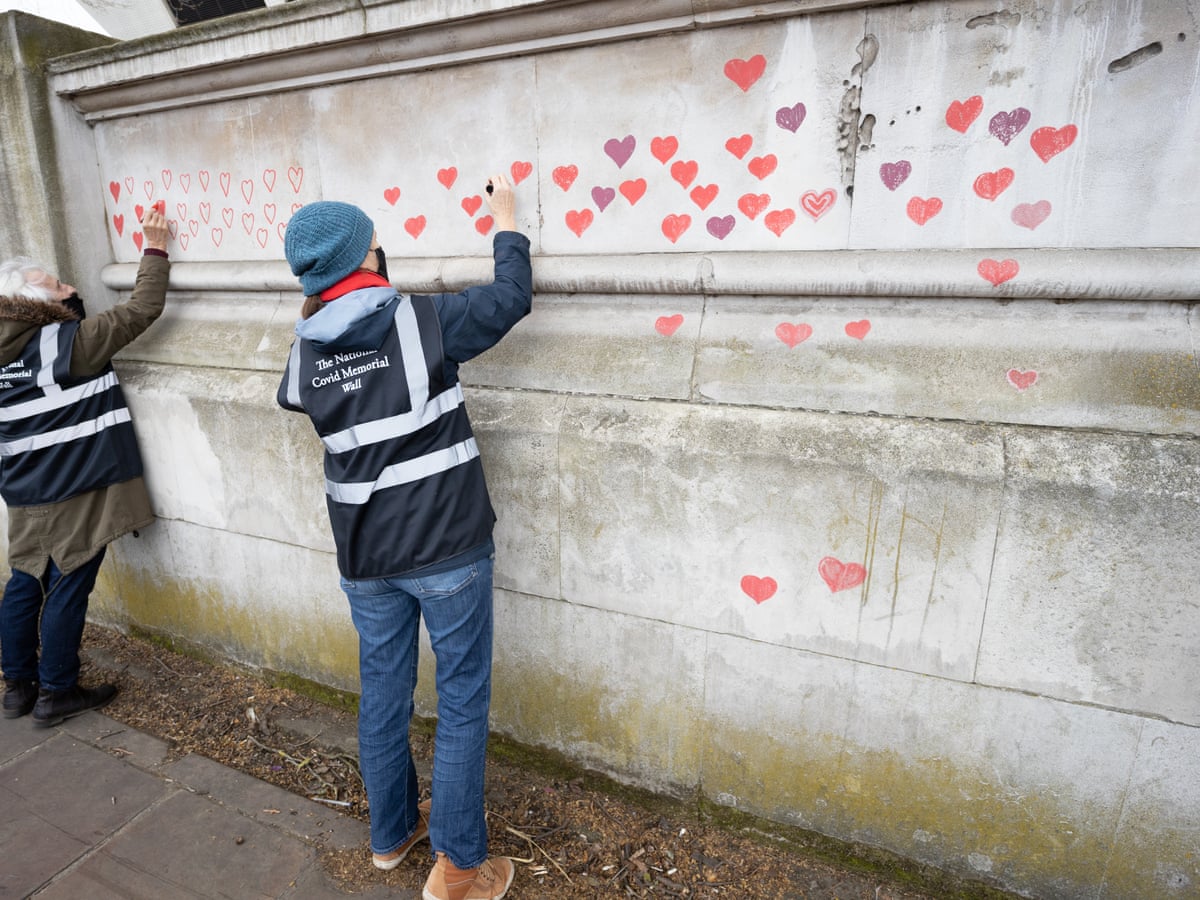The photograph captures two women standing in front of a weathered, gray concrete wall adorned with numerous red and purple hearts. Both women are focused on the wall, filling in hearts with markers. They are wearing black face masks and dark blue jackets with silver reflective stripes, labeled on the back with "The National COVID Memorial Wall." The woman on the right, closer to the camera, is wearing a blue beanie, blue jeans, and light brown shoes. She has her hand against the wall as she draws a heart. The older woman on the far left, who has white-gray hair and is partially out of the frame, is wearing an olive jacket with a fur-lined hood, blue jeans, and dark boots. She is using a red marker to color in the hearts. The memorial wall, approximately 8 feet tall, shows signs of age and grime, and is covered in a mosaic of red and purple hearts, symbolizing the lives affected by COVID-19.